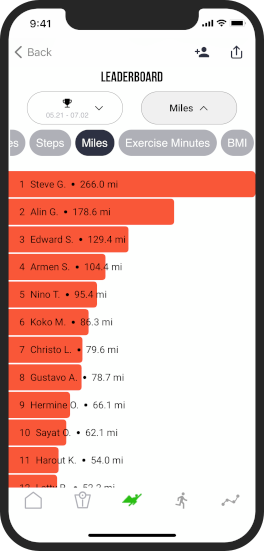The image depicts a cell phone screen showcasing a leaderboard within an exercise tracking app. At the very top, the screen displays the time as 9:41. The app's header features the word "LEADERBOARD" in black, all-cap letters, accompanied by a trophy icon. Just below the header, there's a horizontal rectangular button with rounded edges, highlighted in black, labeled "MILES," indicating the current metric displayed. Other options available for tracking include "STEPS" and "EXERCISE MINUTES," presented in white text against a gray background. 

The leaderboard consists of a ranked list of 12 users, each with their exercise distance in miles. The top three users are Steve G at 266.0 miles, Alain G at 178.6 miles, and Edward S at 129.4 miles. Completing the list are Armin S with 104.4 miles, Nino T with 95.4 miles, Coco M with 86.3 miles, Christo L with 79.6 miles, Gustavo A with 78.7 miles, Hermione O with 66.1 miles, Sia O with 62.1 miles, and finally, Harout K with 54.0 miles. The leaderboard shows individuals' progress in descending order of the distance they have covered.